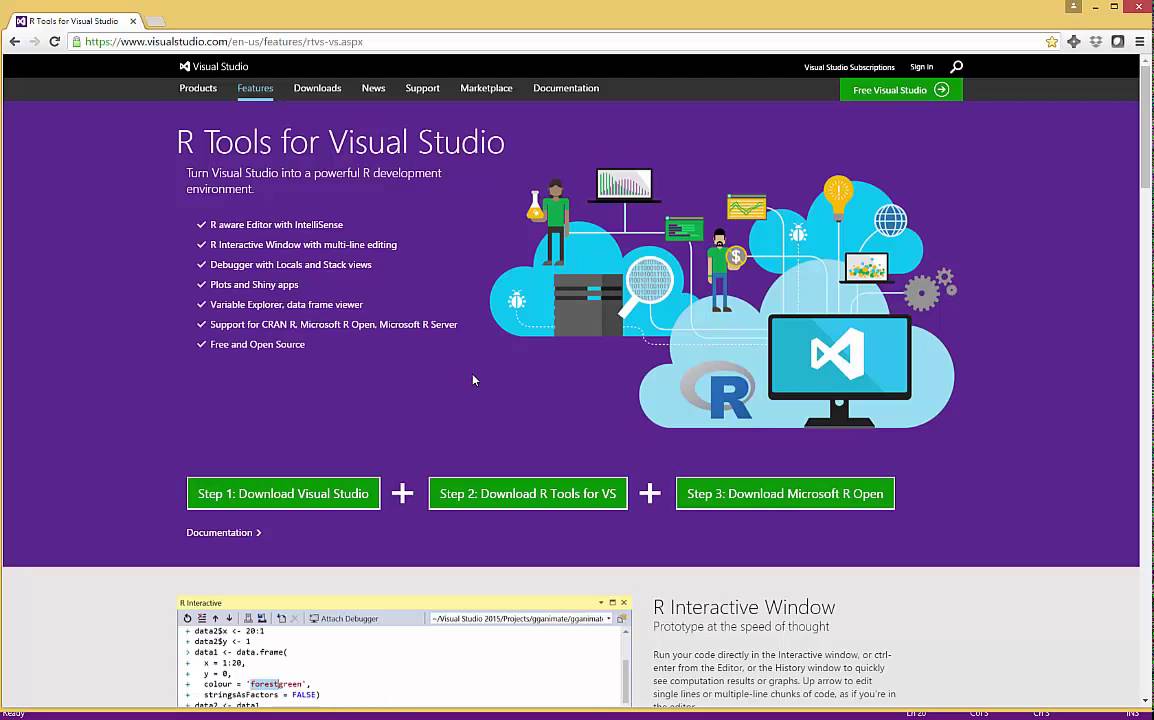Here's a cleaned-up and detailed caption for the described image:

---

The interface displayed shows a webpage with a user interface featuring a yellow border at the top. In the upper right corner, there is a red "X" button for closing the window, along with black minimize and maximize buttons. Beneath this border is a gray tab labeled "Our tools for Visual Studio." Directly below the tab are navigational arrows for back, forward, and refresh, along with an address bar displaying the URL: www.visualstudio.com/en-us/features/rtvs-vs.aspx.

At the top of the webpage, there is a black navigation bar that includes options such as "Visual Studio," "Visual Studio subscriptions," and "Sign in." Below this are additional navigation links: "Products," "Features," "Downloads," "News," "Support," "Marketplace," "Documentation," and a green button labeled "Free Visual Studio," with "Features" being highlighted in blue.

The main page content is titled "Our tools for Visual Studio." The text describes various functionalities, stating: "Turn Visual Studio into a powerful R development environment" and lists features such as:
- R-aware editor with IntelliSense
- R interactive window with multi-line editing
- Debugger with locals and stack views
- Plots and Shiny apps
- Variable explorer
- Data frame viewer
- Support for CRAN R, Microsoft R Open, and Microsoft R Server
- Free and open source

At the bottom of the content are three green download buttons labeled: "Download Visual Studio," "Download R tools for VS," and "Download Microsoft R Open."

---

This caption describes the image comprehensively and organizes the information in a structured manner.